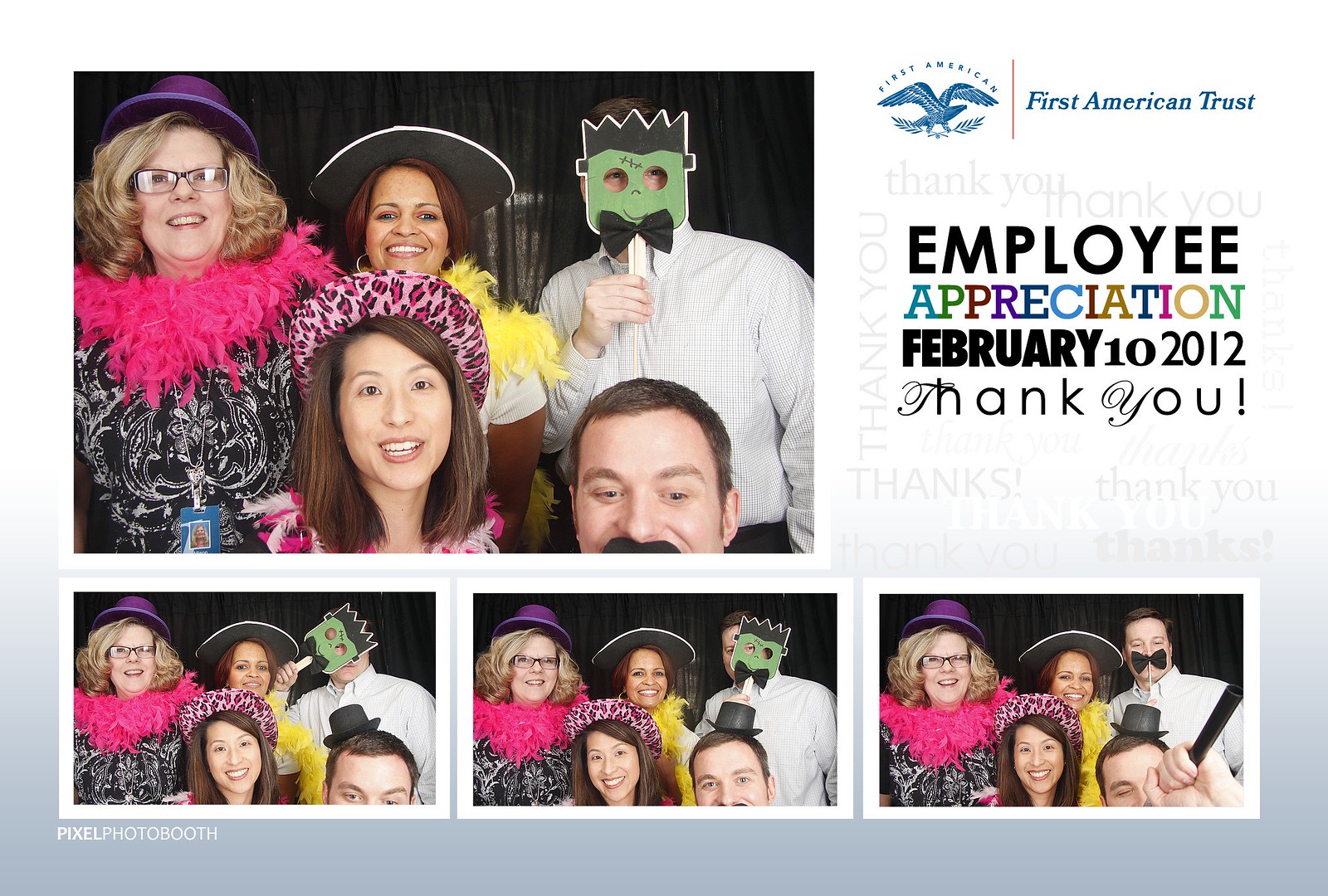The image is a composite of four photos framed by a white-to-grey gradient border. These photos capture a First American Trust Employee Appreciation event held on February 10, 2012. Displayed are three women and two men, all in costumes. One man holds a Frankenstein mask to his face, while the other sports a tiny hat with a large fake mustache. The women wear fancy felt hats in vivid colors—purple, black with a white band, and pink leopard print. Two women also don feather boas, one in pink and the other in yellow. Behind the group is a logo of an eagle, representing First American Trust, and text reading "Employee Appreciation February 10, 2012 Thank You." The photos appear to be taken in a photo booth, with a watermark in the bottom left corner that reads "Pixel Photo Booth." The group is festively dressed, suggesting a celebration, possibly a Halloween party, set indoors.